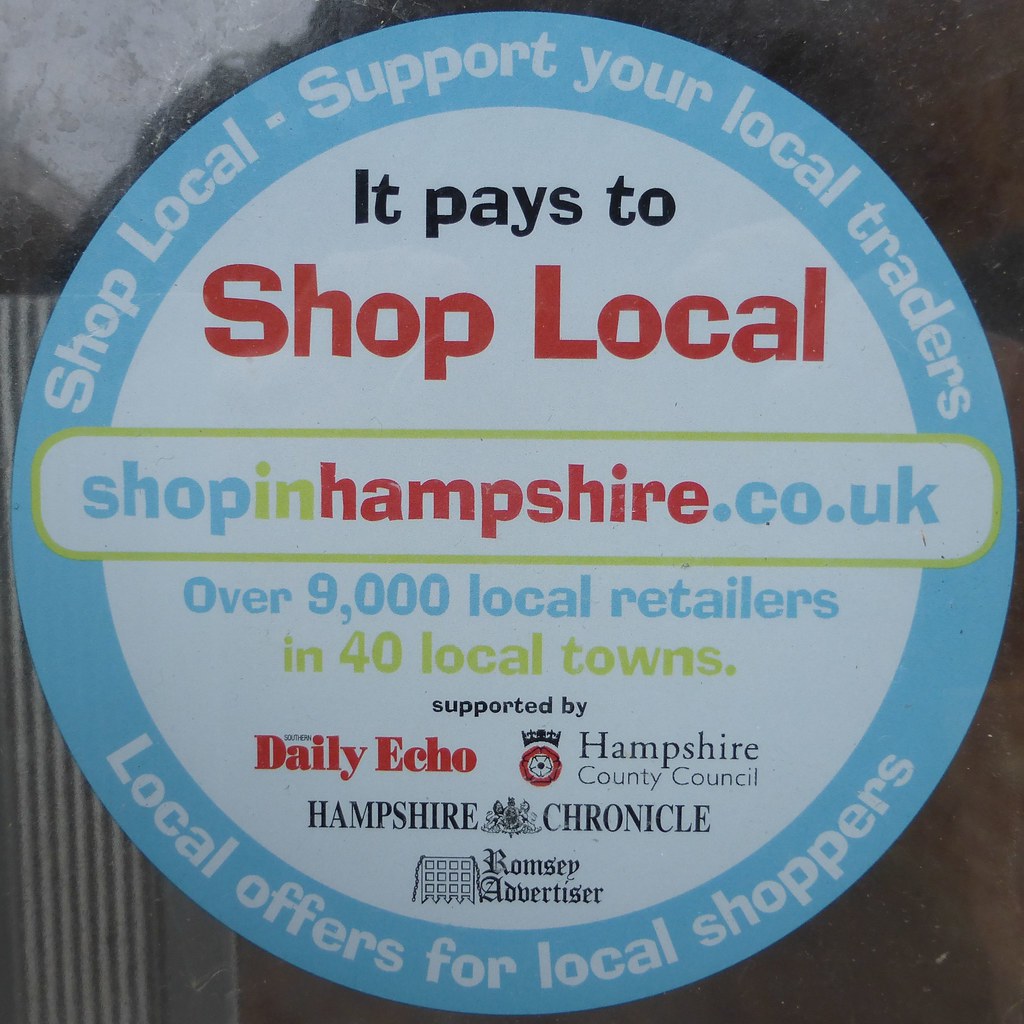The image is a detailed advertisement in the shape of a circle, emphasizing local shopping. The circle features a light blue border with white text along the top and bottom, reading "Shop Local. Support your local traders" at the top and "Local offers for local shoppers" at the bottom. Inside, the circular sign has a white background. Prominently, across the middle, a banner displays the website "Shop in Hampshire.co.uk" in blue, yellow, and red letters with a light green outline. Towards the top within the circle, it states in black and red letters, "It pays to Shop Local." Below the central banner, the text reads "Over 9,000 local retailers in 40 local towns." At the very bottom, the logos of the supporters—Daily Echo, Hampshire County Council, Hampshire Chronicle, and Ramsey Advertiser—are listed, underlining the broad backing for the initiative. The overall message advocates for supporting local businesses and capitalizing on local offers.